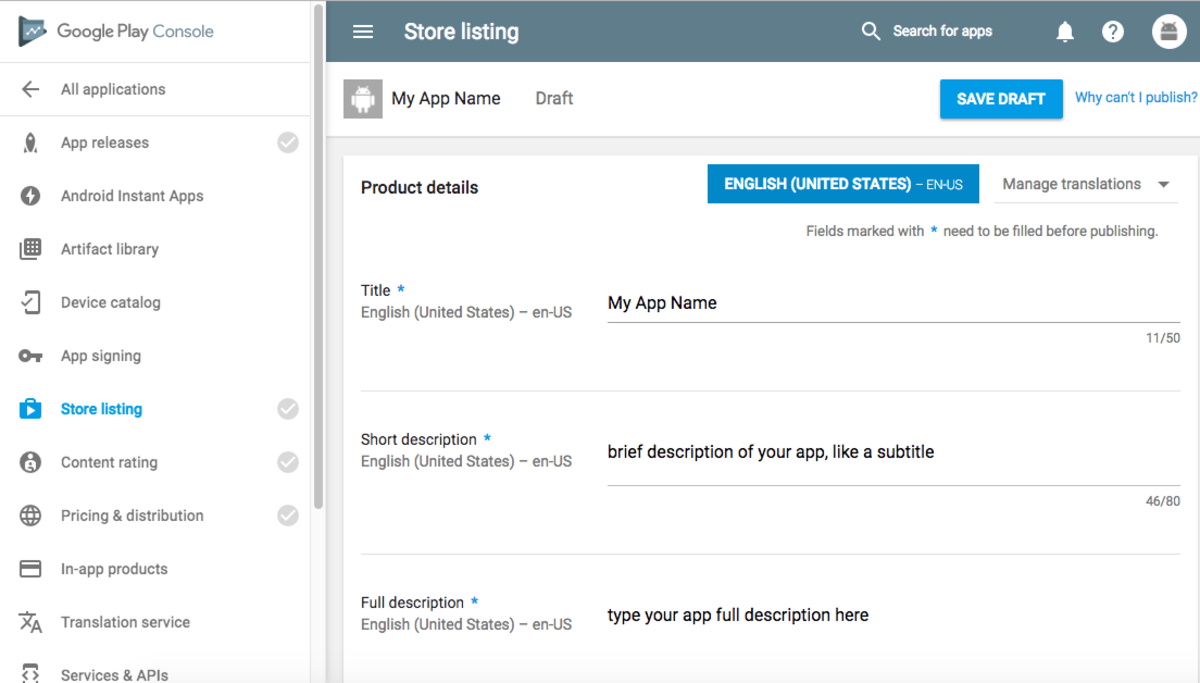In the depicted interface, there is a left-hand sidebar menu titled "Google Play Console." The menu contains various options, including All Applications, App Releases, Android Instant Apps, Artifact Library, Device Catalog, App Signing, Store Listing, Content Rating, Pricing and Distribution, In-App Products, Translation Service, and Services and APIs.

The main webpage section's header features "Store Listing" in the top left corner, accompanied by a menu icon. Adjacent to this is a search bar labeled "Search for Apps," followed by icons for notifications, information, and profile settings. Below the "Store Listing" header, the app's name appears with the notation "draft" next to it.

On the right side of the interface, a prominent blue button labeled "Save Draft" is visible, beside another link titled "Why Can't I Publish?" Below these buttons, the text "Product Details" is displayed, followed by a language indicator "English" and a link to "Manage Translations."

Three sections are provided for text input. The first section, "Title," shows the app's name with a character limit indicator reading "11 out of 50." The second section, "Short Description," prompts for a brief description of the app, with the current input showing "46 out of 80" characters used. The final section, "Full Description," invites users to enter the detailed description of the app.

The arrangement of elements provides a structured layout for managing an app's listing and related details within the Google Play Console.